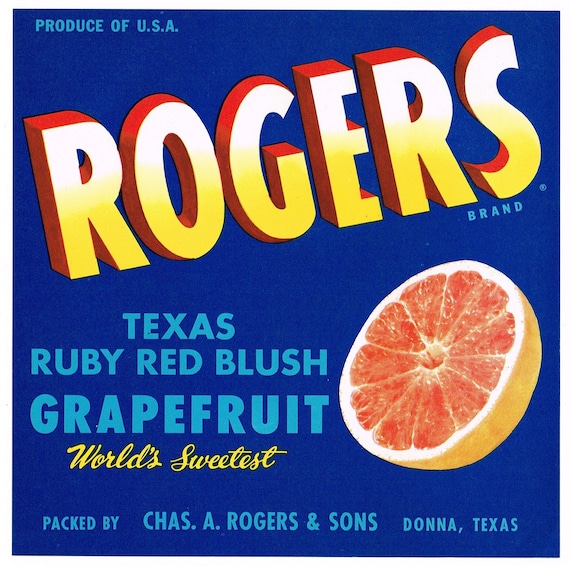The advertisement features a vibrant royal blue background with "PRODUCE OF USA" in light blue, all-caps font in the top left corner. The centerpiece is the "Rogers" brand name displayed in a retro, 3D style font, slanting from the center left to the top right. The letters are outlined and shaded with red, transitioning from white at the top to yellow at the bottom. Below "Rogers," in a centered paragraph format, "Texas Ruby Red Blush Grapefruit" is written in the same light blue, all-caps font, with "Grapefruit" in a larger size. Underneath, "World's Sweetest" is prominently displayed in a gold script font. To the right of the text, there's an image of a half-cut grapefruit, showing its juicy, red interior and a bit of the rind on the right. Across the bottom of the advertisement, "PACKED BY" is written in the lighter blue font, leading to "CHAS. A. ROGERS AND SONS" in a slightly larger size, followed by "DONNA, TEXAS" in smaller text.